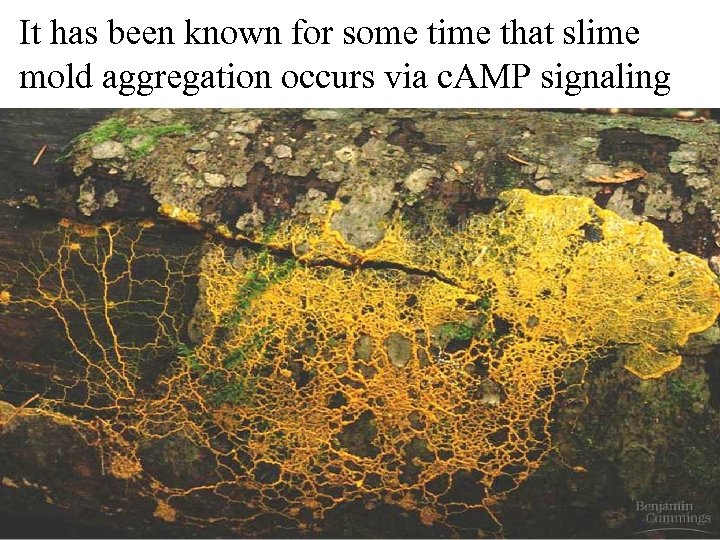This detailed color photograph showcases a yellow slime mold, characterized by its intricate network resembling veins or a sponge, spreading across a rocky surface. The mold aggregation is notable for its vibrant yellow hue and is interspersed with patches of green moss. The rock it grows on transitions from a dark shade at the bottom to a lighter gray at the top, with additional white spots and hints of dried oak leaves visible in the arrangement. The image is labeled with the text, "It has been known for some time that slime mold aggregation occurs via cAMP signaling," with a small "c" and the letters "AMP" capitalized, indicating the biochemical process behind the mold's formation. A reference to Benjamin Cummings is noted at the bottom of the image.